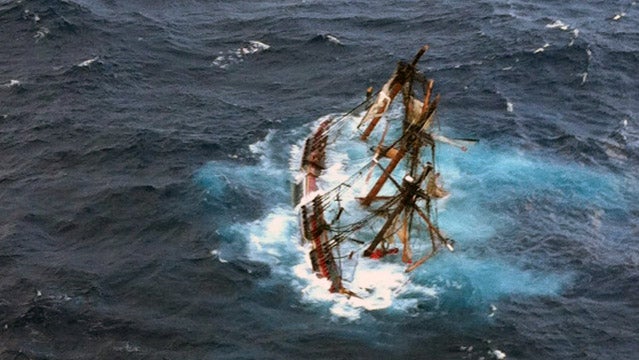This aerial photograph captures a dramatic shipwreck scene, featuring an old wooden galleon-like sailing vessel with three towering masts. The ocean surrounding the ship is a steely gray-blue, accentuated by small white crests on the waves. Contrasting with this, the water immediate to the shipwreck is a bright blue, perhaps due to air bubbles rising to the surface as the vessel takes on water. The ship is angled, tilting towards its port side with the starboard edge partially visible above water, suggesting the hull is nearly submerged. Detailed rigging connects the masts, and a rich red stripe with a gold outline is faintly seen along the top edge of the hull. A mysterious red blob marks the base of the closest mast. This photograph, likely taken from a drone or aircraft, powerfully captures the sinking vessel amid agitated, cresting waves, portraying a moment frozen in time just before the ship disappears beneath the surface.